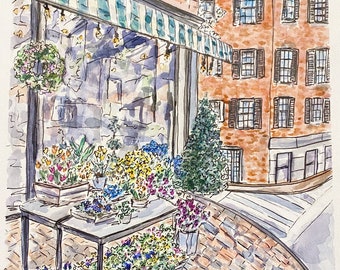This detailed illustration depicts a vibrant corner of a historic city characterized by its distinctive architecture and bustling street scene. On the left side of the image, a quaint flower shop is adorned with an array of colorful flowers displayed on tables outside and hanging baskets overhead. The shop features a charming storefront with a green and white striped awning, giving it a welcoming and lively appearance. The floral arrangements are meticulously placed on black tables with white or glass tops, adding to the shop’s visual appeal.

To the right of the flower shop, a brick building with a classic design captures the eye. This residential building spans three stories, with windows that nearly touch the ground, suggesting that the main floor might be slightly below street level. The use of a combination of markers and colored pencils gives the scene a textured and dynamic look, enhancing both the architectural details and the lush floral displays. The asphalt road separates the flower shop from the residential building, emphasizing the bustling yet harmonious coexistence of commerce and living spaces in this charming urban setting.